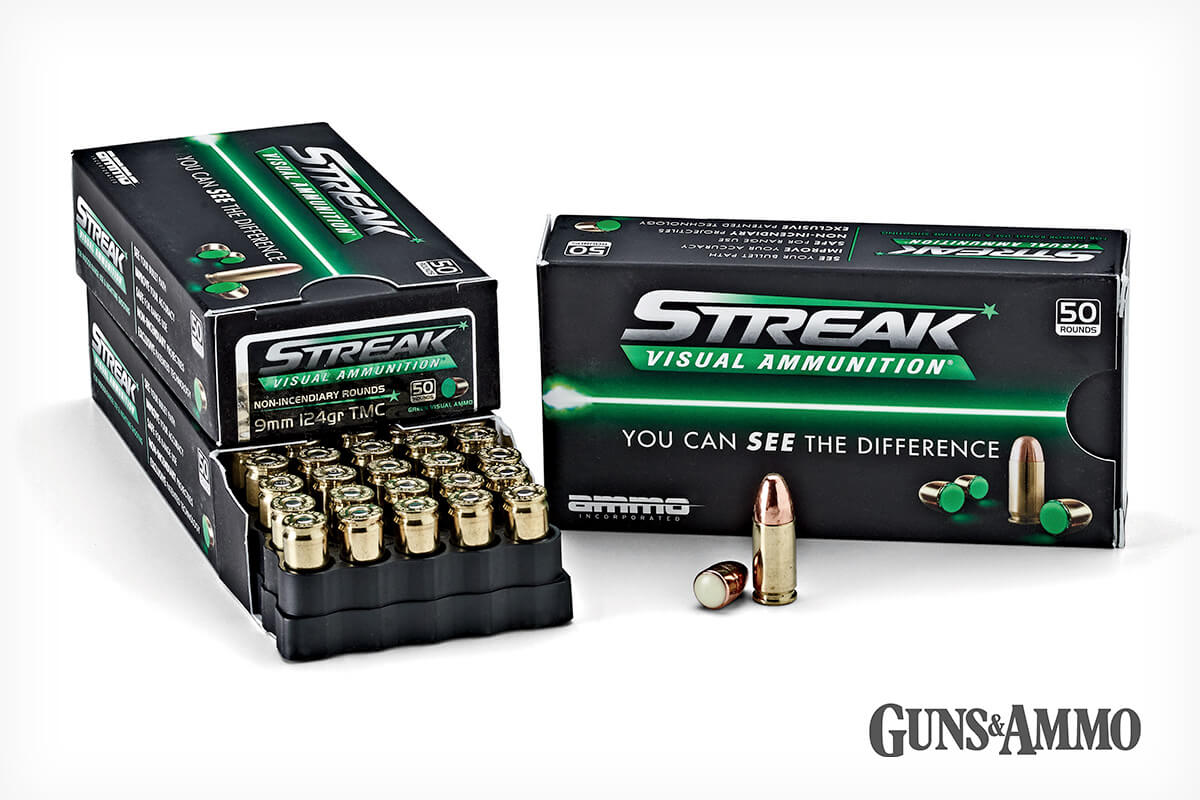The photograph showcases a collection of ammunition displayed against a whitish light blue background. Central to the image is a dark blue box prominently labeled "Streak" in white at the top, accompanied by a green banner reading "visual ammunition." A white streak runs through a blue banner across the middle of the box, and the lower left corner features the word "ammo" in white lettering. 

Positioned to the right of this box, there's another standing box displaying similar branding. In front of it, a metallic gold bullet stands upright while another lies horizontally, revealing its white base. Phrases like "you can see the difference" are inscribed below the green banner, emphasizing the visual distinction of the ammunition.

On the left side of the photograph, two boxes are stacked, with the bottom one slightly pulled out to reveal rows of shiny, gold-colored bullets housed in a black plastic case. The top box also highlights the terms "Streak" and "visual ammunition," and it mentions "50 rounds" in the top right corner. In the bottom right-hand corner of the image, "guns and ammo" is noted in black letters. The bullets, visible throughout the image, exhibit a metallic gold casing with occasional green interior glimpses, accentuating the brand's unique feature.